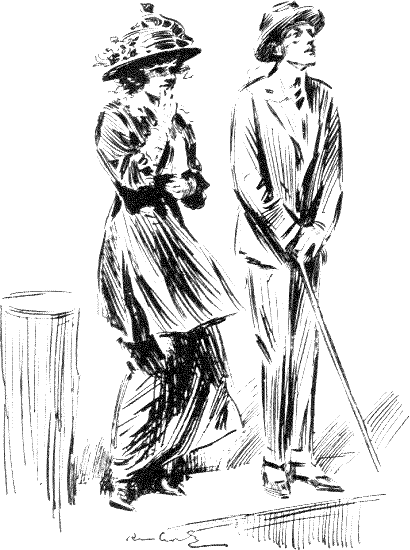This image is a detailed pencil or ink drawing of a middle-aged couple, evocative of the early 20th century, possibly the 1900s to the 1920s. The man, standing to the right, is dressed in a suit with an old-fashioned bowler hat and is holding a cane with his hands crossed in front of him. His shoes are pointed, adding to his formal attire. The woman, standing to his left, is adorned in a long dress that reaches her ankles, with an overlapping skirt or jacket extending to her knees. She wears high-heeled boots or shoes and a large decorative hat embellished with flowers. The woman has one hand raised to her chin and her other hand poised at her waist. Both individuals are looking slightly upwards and to the right, as though observing something intriguing in that direction, such as an aircraft or birds. They appear to be standing on or near a wooden dock, as suggested by the structure to their left. The entire scene is rendered in shades of black and white, and there is a hint of an abstract background, possibly indicating grass. The artist's signature is present but unreadable.